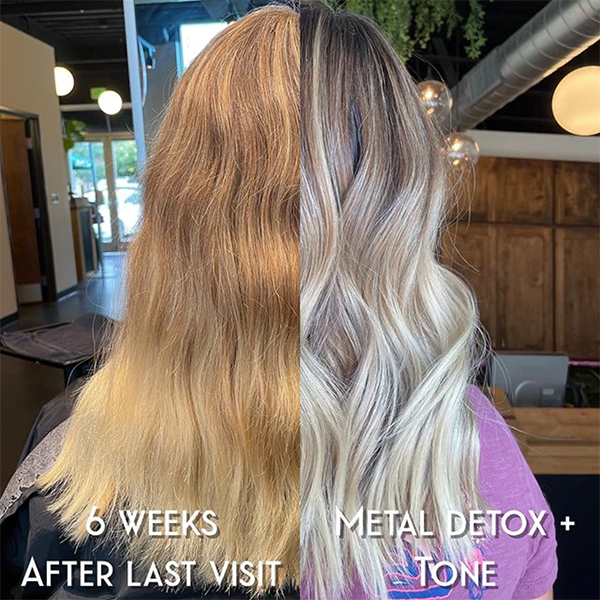The image depicts a split-screen "before and after" comparison of a woman’s hair from the back. On the left side, the text in white capital letters reads "SIX WEEKS AFTER LAST VISIT." The woman's hair appears to be a blend of brown and blonde, with slight reddish tones near the roots. Her hair is relatively straight and shoulder-length. Behind her, there's a hallway with a door and glass doors leading outside, showing daylight. The right side features the text "METAL DETOX PLUS TONE" in white capital letters. Here, the woman's hair is noticeably lighter, almost a grayish-blonde towards the ends and darker at the roots. The hair appears more wavy and separated into distinct strands. The background includes wooden cabinetry, a computer on a table, and metal ductwork visible in the upper right corner.